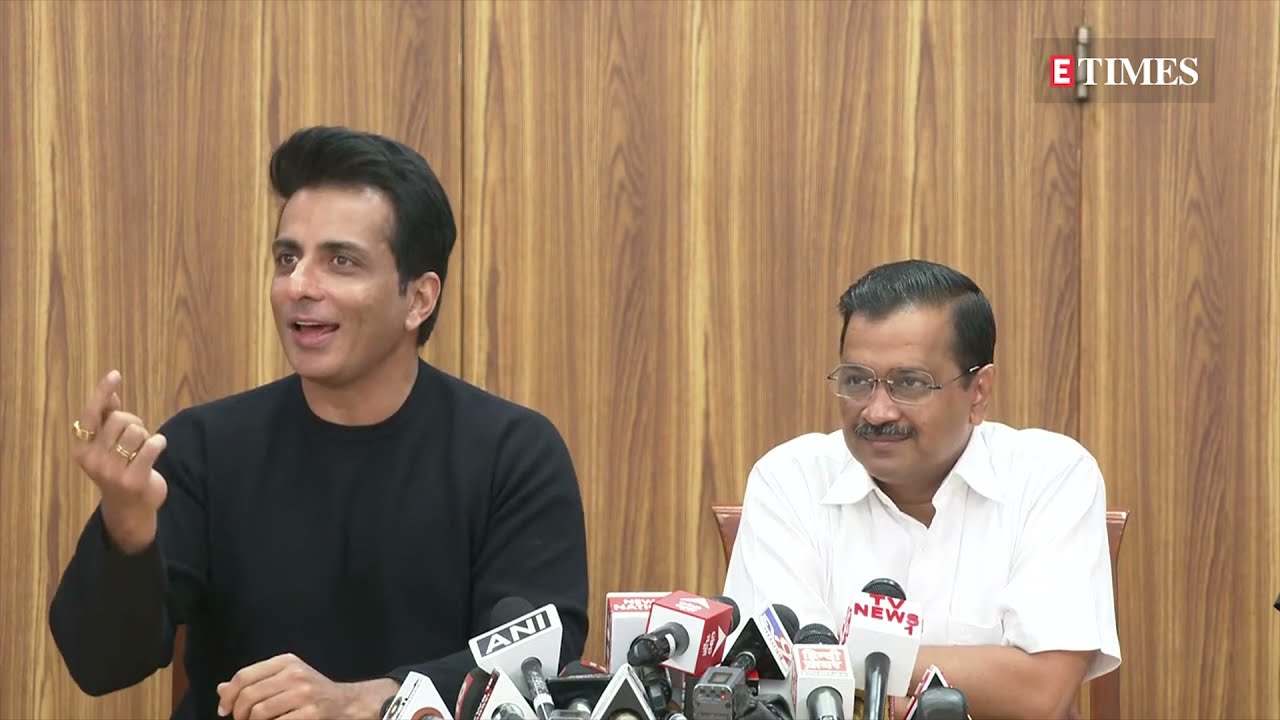In the photograph, two Indian men are seated at a press conference in front of a plain, paneled wooden wall. In the upper right corner of the image, there's a watermark that reads "E TIMES" with a red square containing a white "E" and the word "Times" in white lettering next to it. 

The man on the left, who appears younger, has thick, black hair that's slicked back and raised tall on his forehead. He is clean-shaven and is wearing a black long-sleeved shirt. He is animated, with his right hand raised and a finger pointing upwards, showing two gold rings on his fingers. His mouth is open, as if he is speaking.

Beside him, the older man on the right has slicked-back black hair with some graying, thin wire-framed glasses, and a grayish-brown mustache. He is dressed in a white button-up short-sleeved collared shirt and looks more subdued. Both men are positioned behind a bank of about ten microphones, with one microphone labeled "TV News" in red letters and another labeled "ANI" in black letters.